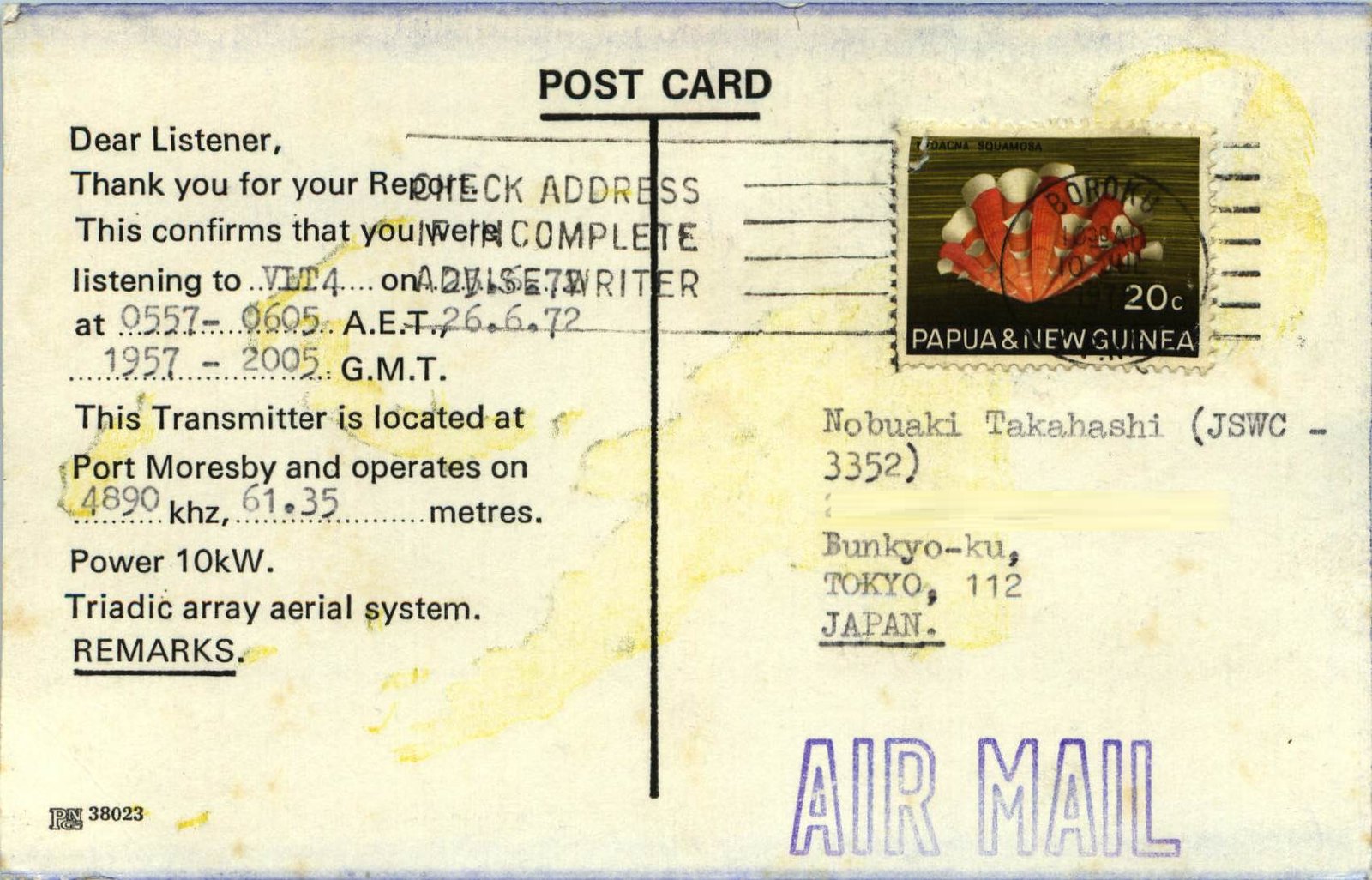The image is of a well-worn postcard, showing significant aging with frayed and bent edges. The white postcard is marred by a large yellow stain in the center. It is divided into two sections by a black line, with "POSTCARD" written in black text at the top center. On the left side, a column of black text begins with "Dear Listener, thank you for your report. This confirms that you were listening to VLT4 at 0557-0605 AET, 157-2005 GMT. This transmitter is located at Port Moresby and operates on 2849 kHz." Additional information includes details about the broadcast frequency, power, and aerial system, some of which is stamped rather than originally printed. On the top right, there's a floral-themed stamp from Papua New Guinea, valued at 20 cents, indicating that the postcard was mailed. Below the stamp appears a blue "airmail" stamp and a return address stating: Nobuaki Takahashi, JSWC 3352 Bunkyoku, Tokyo 112, Japan. The postcard shows visible signs of wear and has multiple stains, emphasizing its age.